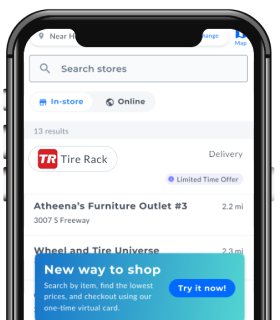The image shows a portion of a mobile phone screen displaying search results within a retail app. At the top of the screen, the search bar contains the text "search stores," and the "in-store" option is selected. Although the exact number of results is unclear, it appears to be either 3.3 or 2.3 results. Prominently, there is a bold red background featuring the white capital letters "T" and "R," adjacent to the text "Tire Rack." The screen also mentions "Delivery" and highlights a "limited time offer." Below this, the search results list "Athena's Furniture Outlet" located 2.2 miles away and "Wheel and Tire Universe" at a distance of 2.3 miles. The lower part of the screen is obscured by a large blue box with white text outlining a new shopping feature: "New way to shop, search by item, find the lowest prices, and checkout using our one-time virtual card." A darker blue clickable area at the bottom states "Try it now."